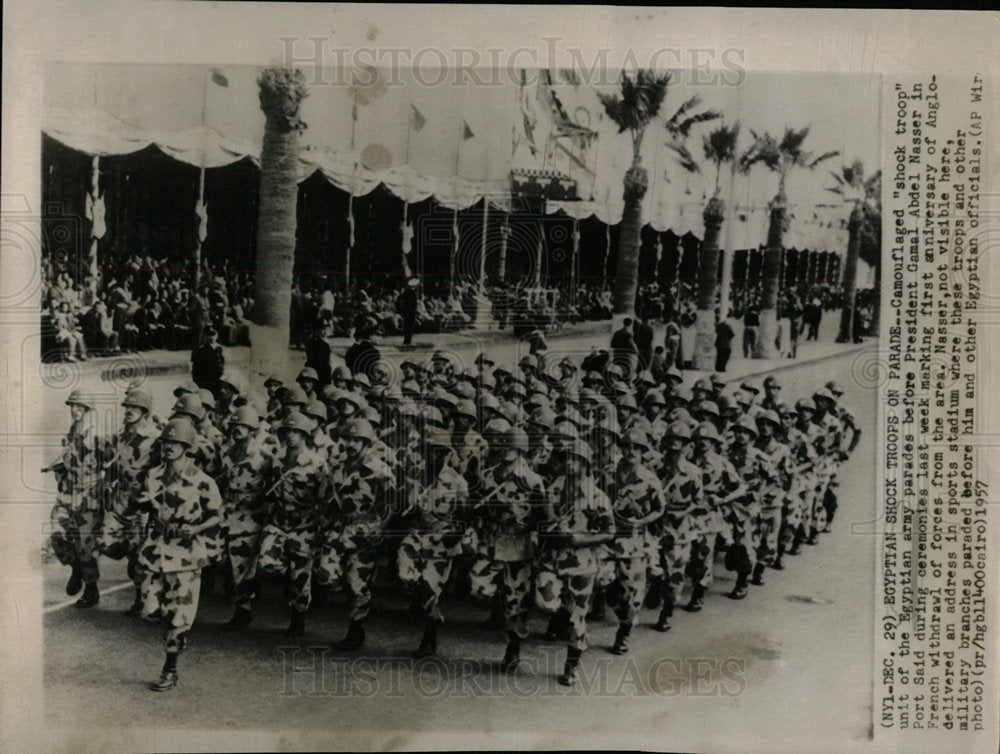This black-and-white historical photograph depicts a significant moment involving the Egyptian military from around 1957. The image shows ten rows of soldiers, all wearing helmets and dark-colored boots, marching forward in a parade formation. Leading them is a solitary figure at the front, distinct from the rows behind him. Superimposed text on the top and bottom reads "historic images." On the right-hand side, additional text details the event: "December 29, Egyptian Shock Troops on Parade. Camouflaged shock troop unit of the Egyptian Army parade before President Gamal Abdel Nasser at Port Said during ceremonies marking the first anniversary of the Anglo-French withdrawal of forces from the area." Though Nasser is not visible in the photograph, the troops paraded before him and other officials, commemorating the completion of the Anglo-French withdrawal.